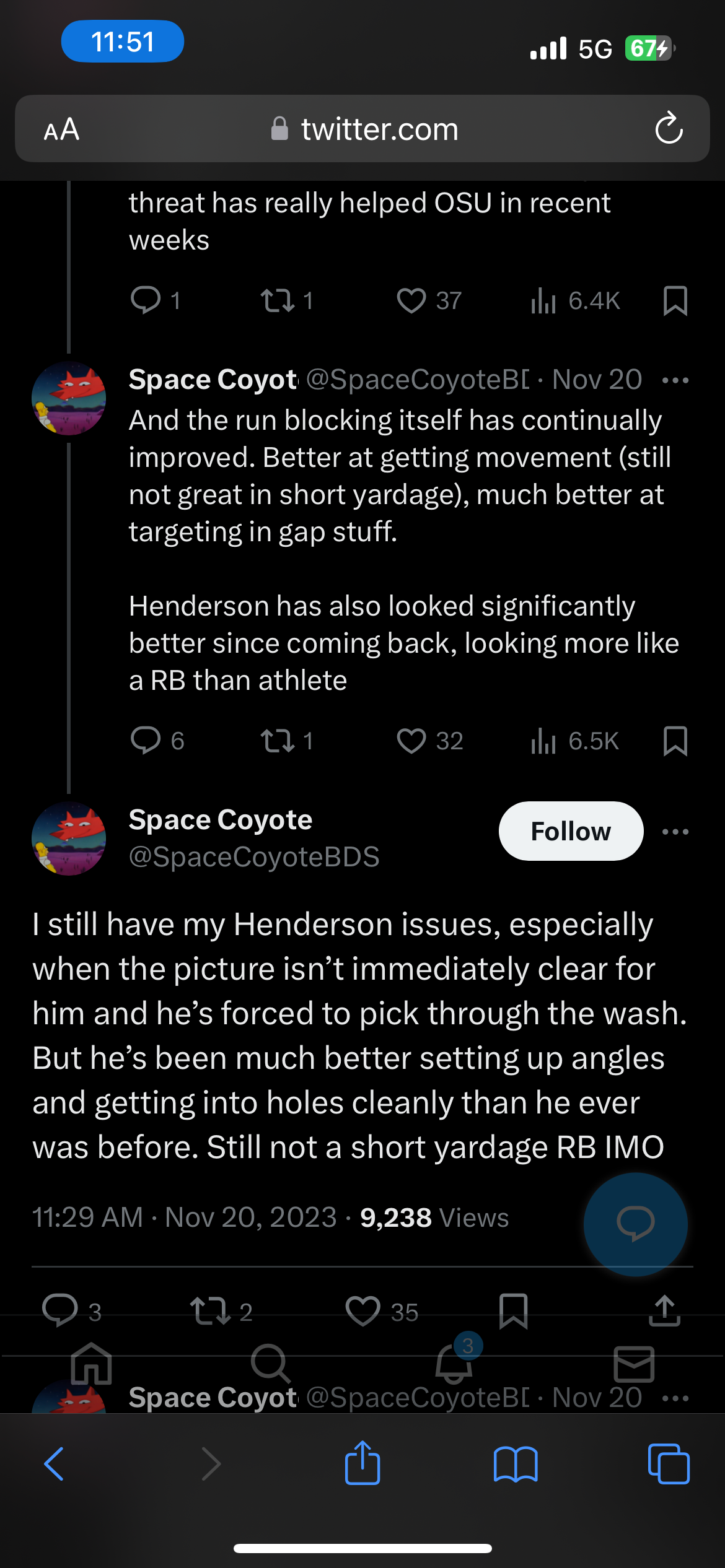This screenshot captures a Twitter feed on a dark mode interface of a smartphone. The background is black, providing a sharp contrast to the white text. 

In the top left corner, the time is displayed as "11:51" in white text against a blue circular background. To the top right, the signal strength is shown with four bars labeled "5G," alongside a battery icon indicating a 67% charge.

The top search bar reads "twitter.com" with a padlock icon for security and a circular arrow icon for page resetting. To the left of the search bar, there are font size adjustment icons represented by a small capital "A" and a larger capital "A."

The feed starts mid-thread with the highlighted tweet exclaiming in capital letters, "THREAT HAS REALLY HELPED OSU IN RECENT WEEKS." The tweet is authored by "Space Coyote," who uses the handle @SpaceCoyoteB, and is dated November 20th. The tweet elaborates, "The run blocking itself has continually improved, better at getting movement (still not great in short yardage), much better at targeting in-gap stuff. Henderson has also looked significantly better since coming back, looking more like an RB than an athlete."

Below that tweet, Space Coyote continues, "I still have my Henderson issues, especially when the picture isn't immediately clear for him, and he's forced to pick through the wash. But he's been much better setting up angles and getting into holes cleanly than he ever was before. Still not a short yardage RB IMO (in my opinion)."